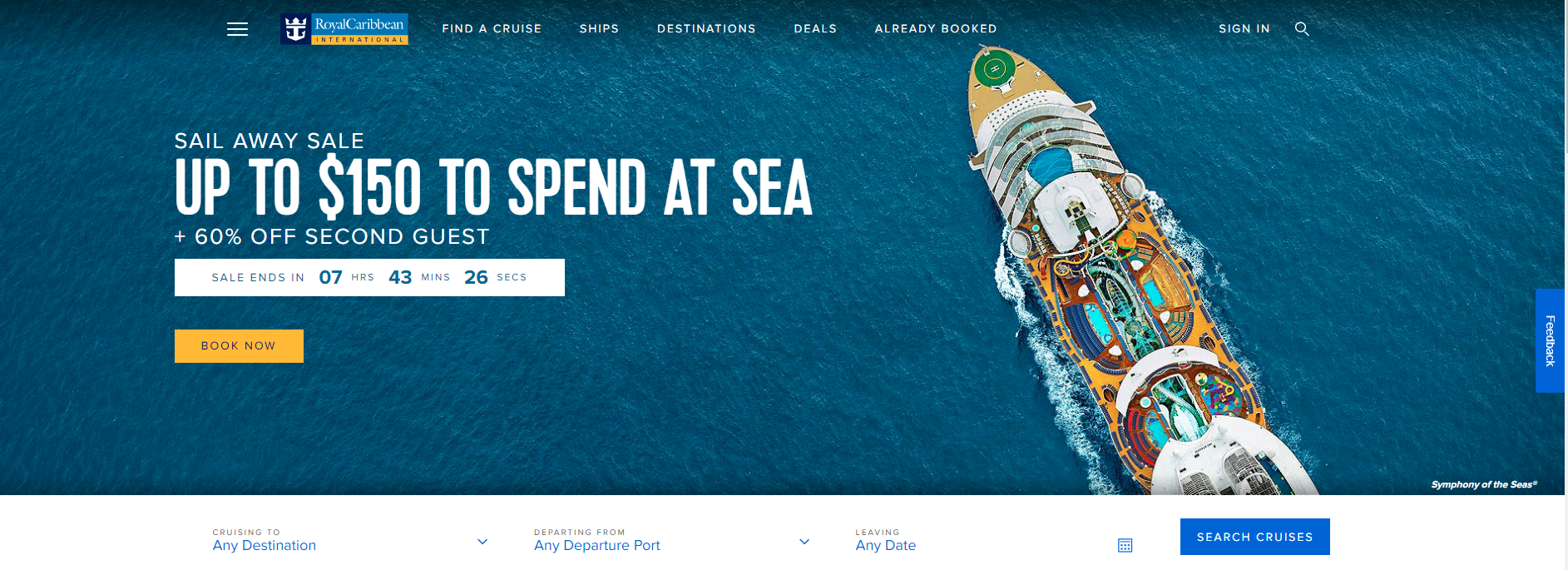The image is a wide website banner, approximately four times as wide as it is tall, showing a top-down view of an aqua blue ocean. The water varies in shades, getting darker towards the edges and lighter at the center. A cruise ship is situated about two-thirds from the left and points diagonally to roughly the 11 o'clock position, leaving a slight wake. The ship is adorned with vibrant orange, yellow, and hints of red and blue.

At the top center of the banner, the Royal Caribbean logo is prominently displayed with the text "Royal Caribbean" next to it. To the right of the logo, menu options read: 'Find a Cruise,' 'Ships,' 'Destinations,' 'Deals,' and 'Already Booked,' followed by sign-in options and a search magnifying glass icon.

Overlaying the center of the image, bold white text announces a "Sail Away Sale." Below it, in large font, the promotion "Up to $150 to spend at sea" is highlighted, with a smaller text beneath it offering "Plus 60% off second guest."